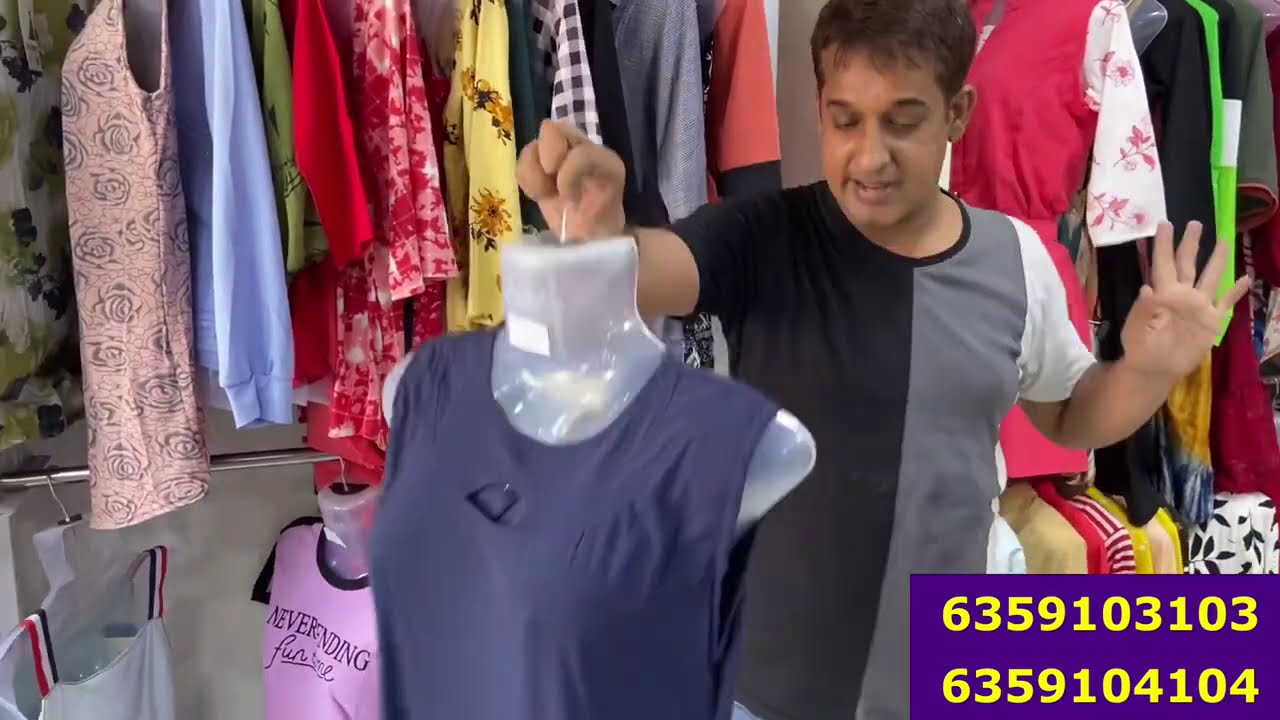In this close-up, full-color photograph taken indoors at a clothing shop, a man with darker skin—perhaps of Indian, Middle Eastern, or Hispanic descent—stands in front of two rows of colorful clothes. These racks display a variety of tops, including sleeveless, short sleeve, and three-quarter sleeve shirts in multiple hues, such as pink, blue, green, red, yellow with floral patterns, and black-and-white checkered designs. There is also a dress to the right of the man. He wears a black, gray, and white short-sleeved t-shirt, has dark short hair with a few bangs on his forehead, dark eyebrows, and an open mouth while looking down. His left hand is raised at his side, and his right hand is stretched forward, holding part of a mannequin that wears a blue sleeveless shirt. In the lower right corner of the image, there is a purple rectangular box with yellow numbers: 6359103103 and 6359104104.